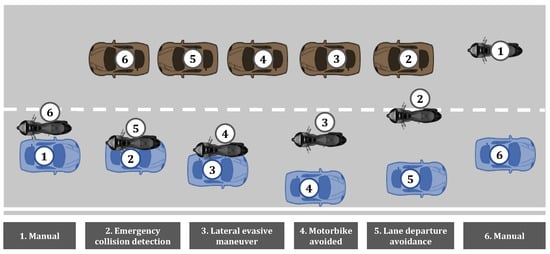The image is an overhead, illustrated diagram of a street depicting traffic flow and collision avoidance systems. On the upper lane, which moves to the left, there are five brown cars numbered two through six, followed by a black motorcycle labeled number one. On the opposite bottom lane, moving to the right, there are six cars and five motorcycles in different positions relative to each other, with the motorcycles facing oncoming traffic. Beneath the image, gray rectangles with white text provide explanations for the numbers, including terms like manual, emergency collision detection, lateral evasive maneuver, motorbike avoided, lane departure avoidance, and manual. This setup suggests it is likely for educational purposes, possibly related to driver safety and collision detection systems.